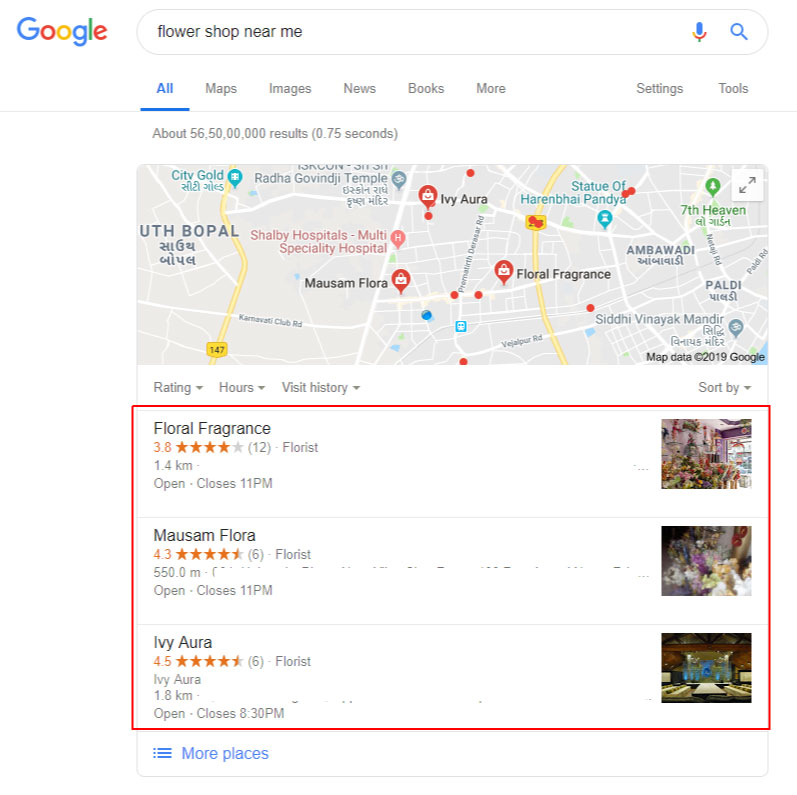In the top left corner of the image, the Google logo is prominently displayed, with each letter in a distinct color: the first 'G' in blue, the first 'O' in red, the second 'O' in yellow, the second 'G' in blue, the 'L' in green, and the 'E' in red. The search query "Flower Shop near me" is entered in the search bar with a microphone icon and a magnifying glass icon on the top right side of the search bar.

Below the search bar, navigation options are visible, which include "All," "Map," "Images," "News," "Books," "More," "Settings," and "Tools." The search results indicate approximately 56,500,000 results found in 0.75 seconds.

The initial search results feature a list of flower shops with brief descriptions:
1. "Floral Fragrance" with a rating of 3.8 stars, located 1.4 KM away, with opening hours until 11 PM.
2. "MAUSAM Floral" with a rating of 4.3 stars, located 550 meters away, also open until 11 PM.
3. "Ivory Zora," appearing twice for clarity, with a rating of 4.5 stars, located 1.8 KM away, with opening hours until 8:30 PM.

Accompanying the search results, map pinpoints indicate the locations of these flower shops along with thumbnails of flower shop images.